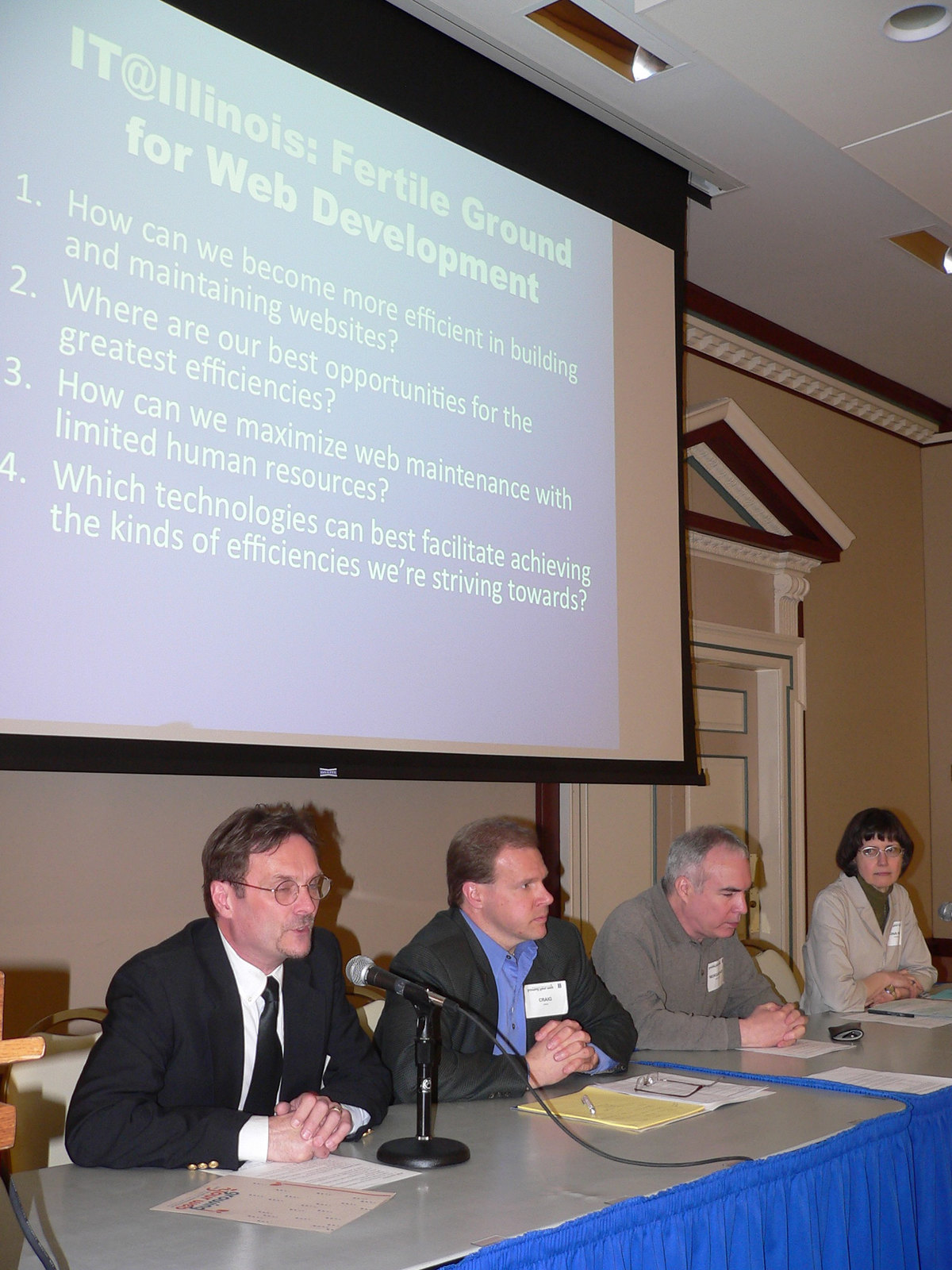In the image, a meeting or seminar is in progress, likely a focus group, taking place in a room with two tables draped in blue skirting in the foreground. Four individuals are seated in a row behind these tables. The first man on the left, wearing a suit and tie with glasses, is speaking into a microphone with his hands folded. Next to him is another man dressed in a blue shirt and black blazer, also with a white name tag and leaning forward with his hands folded. An elderly man with gray hair, sporting a white name tag, gazes downward pensively. At the far right, a woman in business attire attentively listens to the speaker. 

Behind them, a large PowerPoint slide is projected on a screen, featuring a blue background with white text under the header "IT at Illinois: Fertile Ground for Web Development." The slide lists four discussion points: 
1. How can we become more efficient in building and maintaining websites?
2. Where are our best opportunities for the greatest efficiencies?
3. How can we maximize web maintenance with limited human resources?
4. Which technologies can best facilitate achieving the kinds of efficiencies we're striving towards?

The room's ambiance suggests a formal setting focused on addressing critical questions related to web development and efficiency, indicated by the list on the presentation. Papers are scattered on the white surface of the tables, and a doorway is visible on the right side of the image, adding to the setting's context.